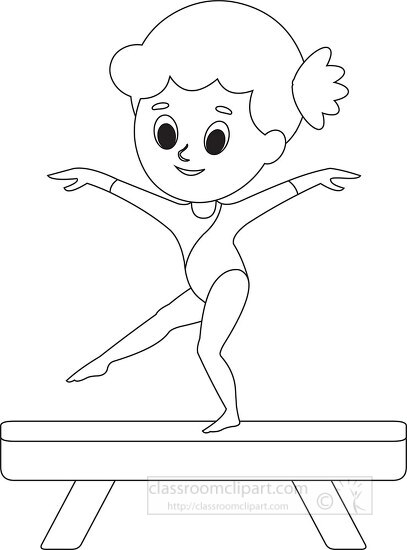This detailed cartoon drawing, reminiscent of a coloring page, features a young gymnast elegantly balanced on a beam. She stands confidently on her left leg, with her right leg extended gracefully behind her, toes pointed. Her arms stretch out to either side, fingers splayed in a claw-like fashion due to the artistic style. A delicate ponytail adorns the left side of her head, complementing her visible left ear. Her expressive face displays large eyes with prominent black ovals surrounded by a hint of white, eyebrows curved like upside-down question marks, and a small nose. Her mouth forms a cheerful smile, suggesting the presence of teeth. She wears a form-fitting leotard, accentuated by a stripe running from her neckline diagonally across to her side. The overall scene captures the poise and concentration of the gymnast in mid-performance.